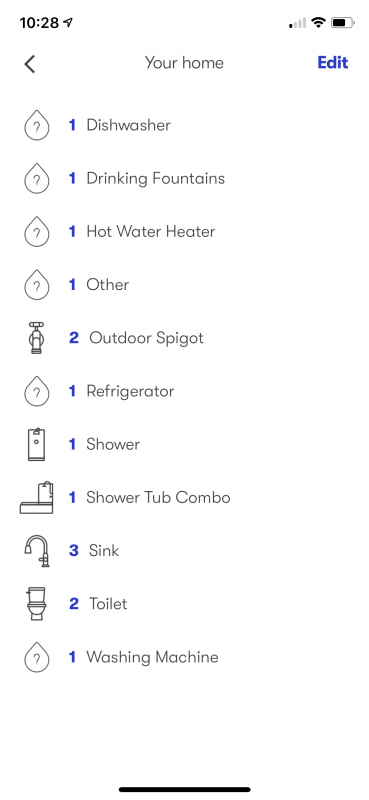Screenshot of a mobile website displaying home features with icons:

The screenshot, taken at 10:28 AM, showcases a mobile site with a single cellular signal bar, full Wi-Fi signal, and a half-full battery icon. At the top, the header reads "Your Home" alongside a blue "Edit" button. Below the header, there's a detailed list of home features each accompanied by a representative icon. The inventory includes: one dishwasher (icon of a dishwasher), one drinking fountain (icon of a fountain), one hot water heater (icon of a water heater), one item labeled as "other" (unidentified icon), one outdoor spigot (icon of a spigot), one refrigerator (icon of a fridge), one shower (icon of a showerhead), one shower-tub combo (icon of a bathtub with a showerhead), three sinks (icon of a sink), two toilets (icon of a toilet), and one washing machine (icon of a washing machine). The icons make it easy to identify each item at a glance.